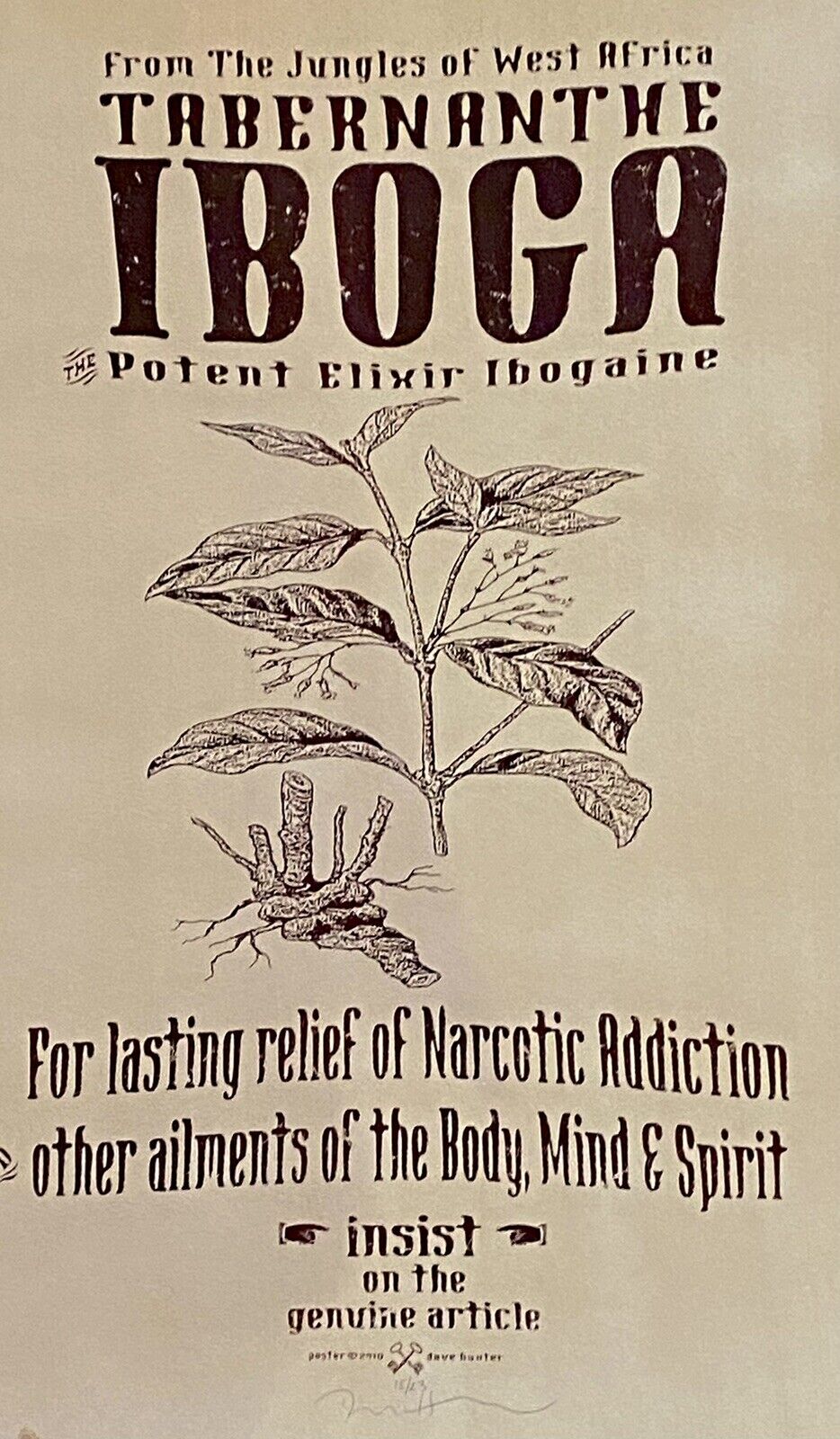This advertisement, printed on a tan piece of paper using dark brown font, showcases an old, likely vintage, promotion for a product called Tabernanthe Iboga. At the top, it declares "From the jungles of West Africa, Tabernae Iboga, Potent Elixir Ibogaine." In the center, there is an intricate illustration of the Iboga plant, featuring pointy, undulating leaves and net-like flowers on either side. Below the plant, the text emphasizes, "For lasting relief of narcotic addiction and other ailments of the body, mind, and spirit. Insist on the genuine article." Notably, the word "insist" is highlighted with pointing fingers on either side. The advertisement appears to be signed at the very bottom, giving it an authentic and antique feel.